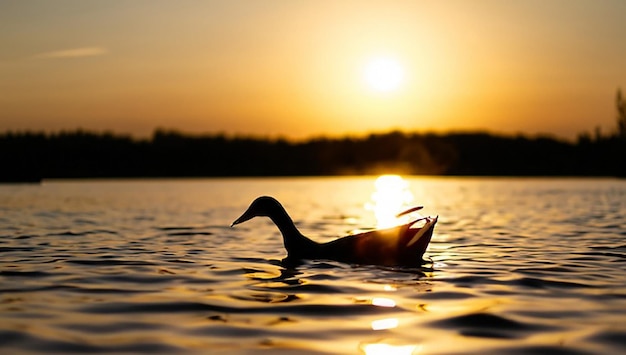In the foreground of this image, a solitary duck with its head facing left swims gently on a large lake, creating light ripples around it. The duck appears mostly as a dark silhouette, though some sunlight catches its feathers, highlighting them slightly. The water itself is a darker hue, with reflections of the sun twinkling on its surface. The sky above displays a vivid orange, indicating this scene is captured at sunrise. The sun is just above the horizon, casting a warm glow and reflecting off the water. In the background, a dense area of greenery and perhaps mountainous terrain is discernable despite the low light. One small cloud floats in the otherwise gray sky, contributing to the serene and tranquil atmosphere. On the left side of the image, a boat can be faintly seen, adding a subtle detail to the picturesque scene.